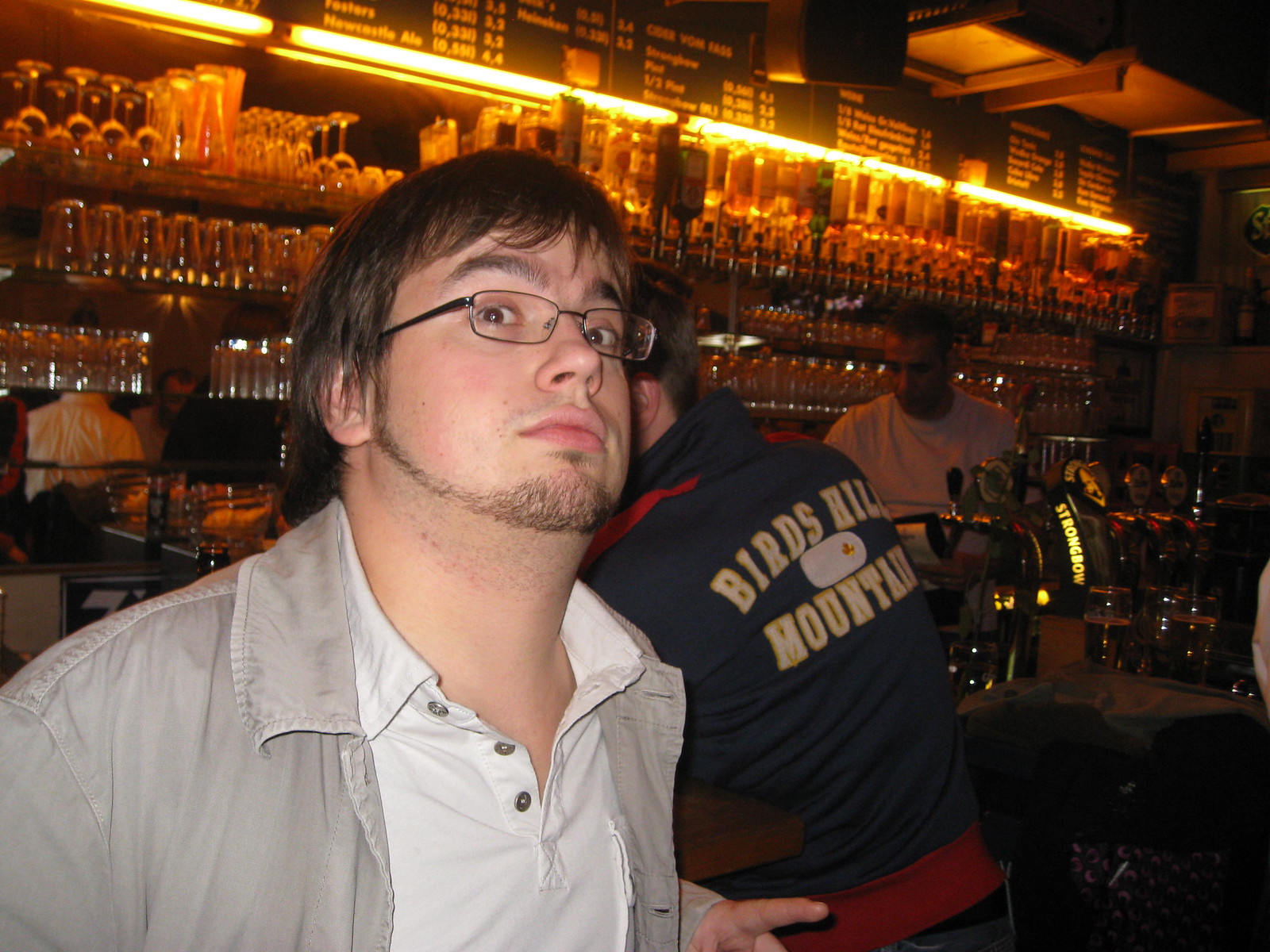The photo is set inside a dimly lit, cozy bar. The focal point is a young man in his mid-20s, positioned on the left side near the center of the image. He looks surprised as he stares forward with his head slightly tilted up. He sports a shaggy hairstyle that falls over his ears, a thin chin-strap beard with a soul patch, and wears glasses with black frames. His attire includes a white polo shirt under a light grey jacket.

In the background, the bar features a warm, brownish-yellow ambiance with light emanating from bulbs atop a shelf filled with a variety of glasses. The neatly arranged glassware and multiple beer taps hint at a well-maintained establishment. To the right, a man in a black jacket with white designs on the shoulders faces the bar, with the words "Bird's Hill Mountain" visible on the back of his blue hoodie. A bartender in a white T-shirt stands behind the bar, attending to tasks, adding to the lively yet relaxed setting of this upscale bar.